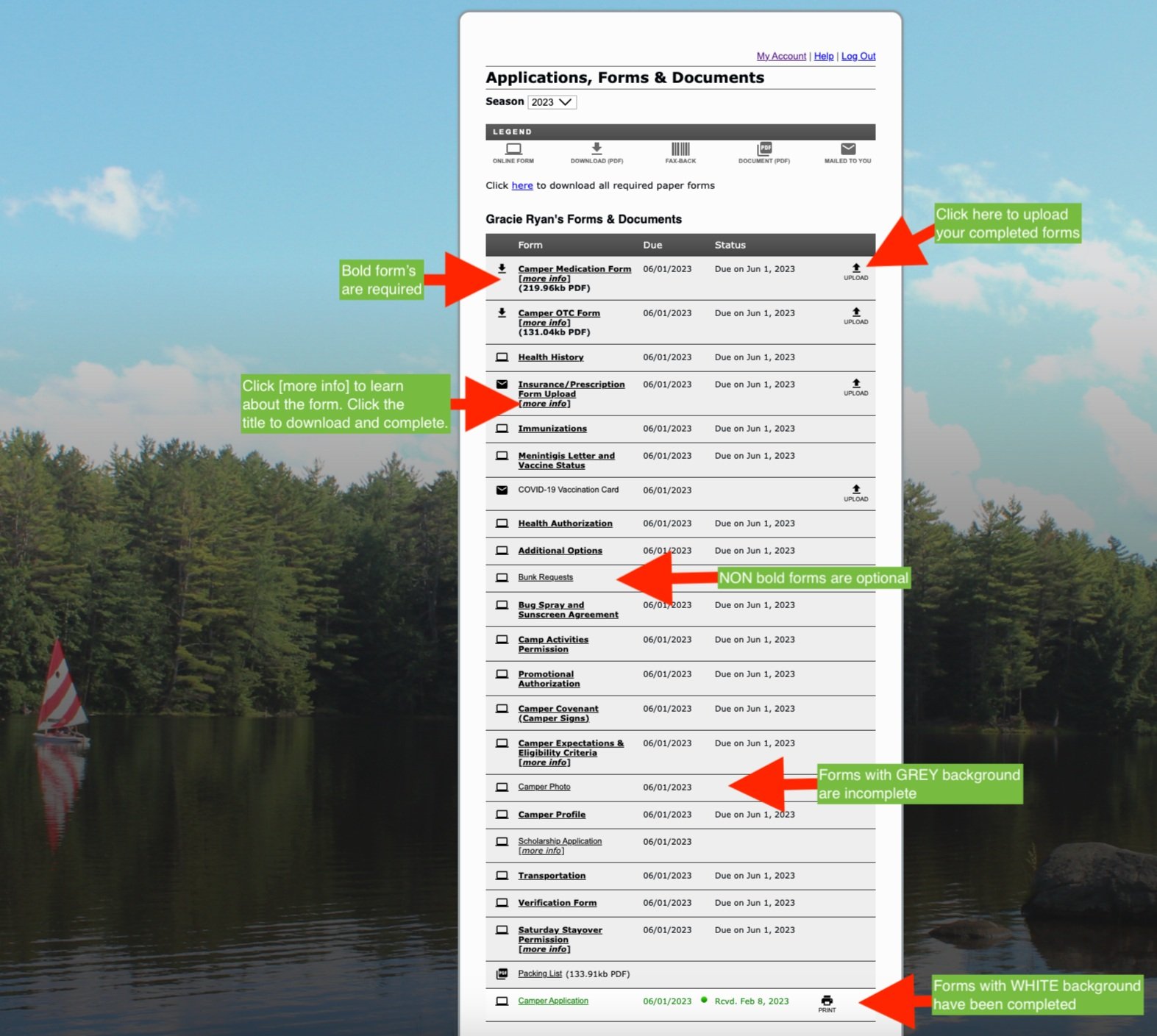This image captures a serene outdoor scene featuring a picturesque pond or lake under a bright sky, where blue hues blend harmoniously with fluffy white clouds. In the background, lush green trees provide a charming natural frame. Centered on the water is a sailboat adorned with striking red and white stripes, creating a vivid focal point. The sailboat’s reflection is beautifully mirrored in the clear water, adding a sense of tranquility. Additionally, a large rock juts out from the water’s surface, adding texture to the landscape.

On the right side of the image, there is an overlay consisting of a box labeled "Application Forms and Documents," accompanied by numerous red arrows. Each arrow points to specific spots on the underlying image, with green rectangular boxes attached to them containing text. Due to the small font size, the text within these boxes is mostly unreadable, though sporadic words like "click" and "download" can be discerned. The overall juxtaposition of this informative overlay with the serene natural scene creates an intriguing contrast.